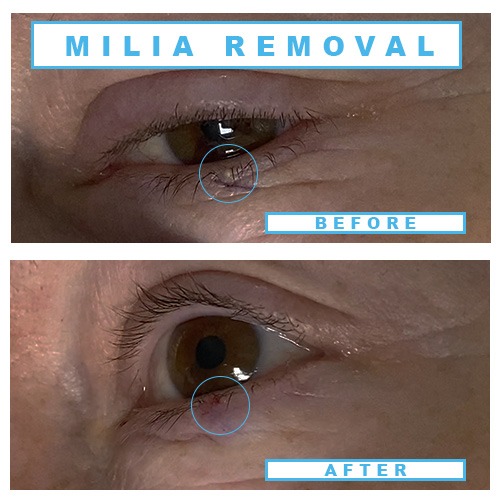The image consists of a detailed before-and-after comparison of a close-up view of a Caucasian person's eye, highlighting a milia removal procedure. At the top, within a blue rectangular box featuring white background and blue lettering, the words "MILIA REMOVAL" are displayed prominently. Below this text is an image of the eye with a blue circle around the lower eyelid area. Inside the circle, the word "BEFORE" is printed in blue lettering on a white background. This initial image shows the eye partially open with light brown pupils and the presence of milia.

In the lower part of the image, a more magnified view of the same eye is presented, this time fully open. The eye appears to be slightly watery, and within the blue circled area, a small red spot with minor bruising is visible, indicating the site of milia removal. Below this closer image, the word "AFTER" appears in blue lettering on a white background, also within a blue rectangular box. The layout and the context emphasize the changes post-procedure, offering a clear visual contrast between the conditions of the eye before and after milia removal.